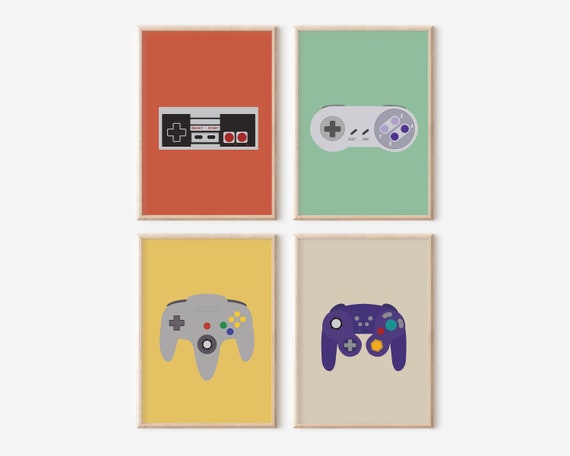The image features a series of four framed artworks, arranged in a checkerboard pattern, each one showcasing a different generation of Nintendo controllers. The frames are made of light pine wood, adding a simple yet elegant touch to the display. 

Starting in the upper left, set against a coral red background, is the iconic rectangle-shaped NES controller. This classic controller features a D-pad on the left, start and select buttons in the middle, and two red action buttons on the right.

Moving clockwise, the second artwork is set against a seafoam green background and displays the Super Nintendo controller. It is a more rounded design with a similar layout: a D-pad on the left, start and select buttons in the center, and the distinctive purple and lavender action buttons on the right, complemented by shoulder buttons.

Continuing to the bottom right, on a sandy beige background, is the Nintendo 64 controller. This gray controller stands out with its unique three-pronged design, an analog stick in the center, a red start button, and differently colored blue, green, and yellow buttons, along with a traditional D-pad and shoulder buttons.

Finally, in the bottom left, with a mustard yellow backdrop, is the GameCube controller. This purple controller introduces two analog sticks along with the D-pad, start button, and a range of action buttons labeled A, B, X, and Y, as well as shoulder buttons.

These artworks collectively represent the evolution of Nintendo controllers, from the NES to the GameCube, each set against a distinct pastel or solid colored background, perfect as wall art for a gaming room.